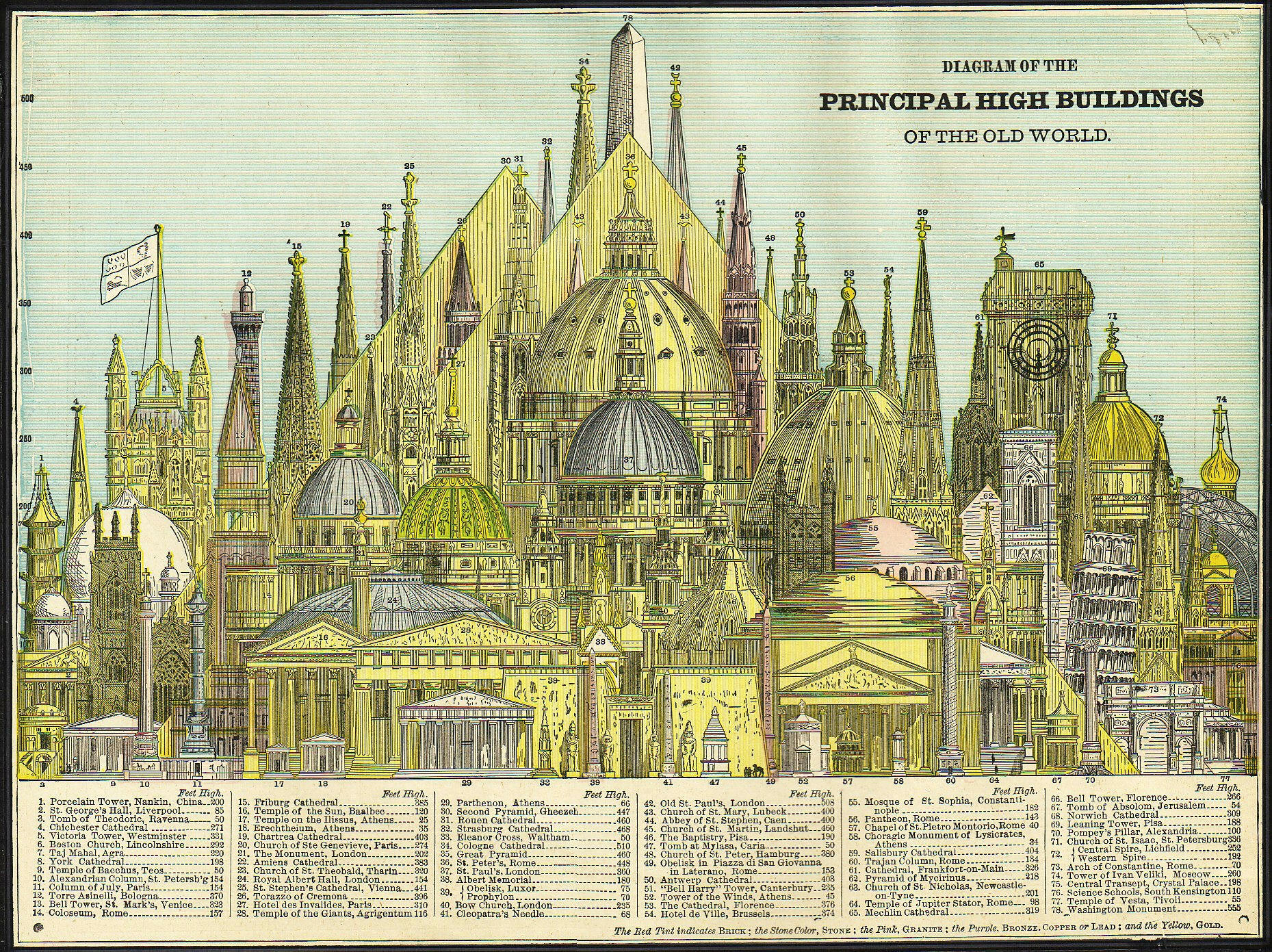A captivating vintage poster titled "Diagram of the Principal High Buildings of the Old World" showcases a detailed illustration of architectural marvels from across different regions. The diagram is segmented into six categories, displaying an array of notable structures, some highlighted in black and yellow while others remain in pure black ink. Dominating the layout, yet meticulously small in print, the poster features iconic edifices such as the Leaning Tower of Pisa—standing modestly shorter than its towering counterparts—and a multitude of cathedral towers and domes. Among these, St. Paul's Cathedral and potentially one of Moscow's famed cathedrals make an appearance, yet their labels are difficult to discern without a magnifying glass or exceptional eyesight. Each structure is methodically numbered, awaiting the keen observer's discovery.